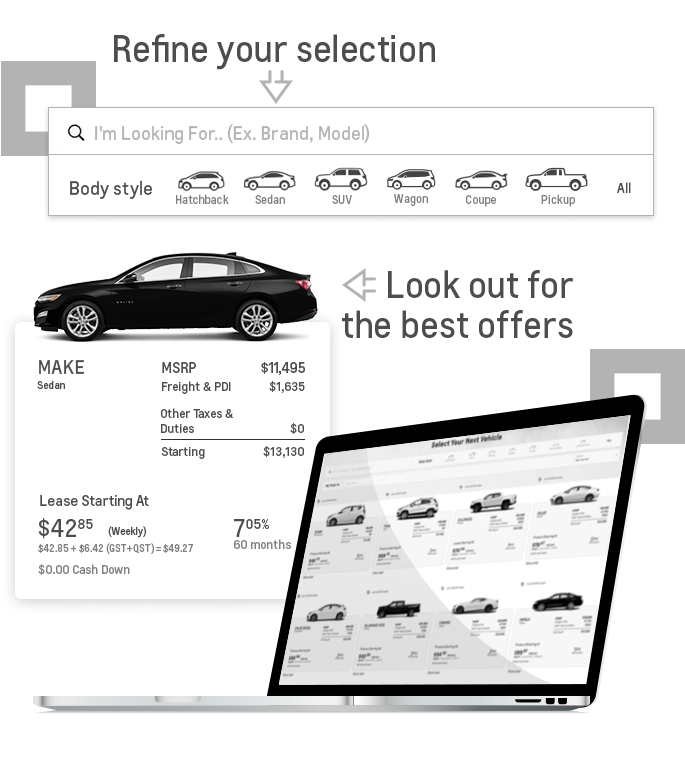The image features a clean, white background with a central gray square outlined. At the top of the square, there is a search bar labeled "Refinder Selection" with a down arrow for options. The search bar categories include body styles: hatchback, sedan, SUV, wagon, coupe, pickup, and a choice for "All." Displayed prominently is a sleek black car with a call-to-action message, "Look out for the best offers," accompanied by a left-pointing arrow.

Further details include the car's pricing information: the MSRP is set at $11,495, with additional charges for Freight and PDI at $1,635 (PDI in capital letters). There are no other taxes or duties, bringing the starting price to $13,130. Leasing options are also highlighted, starting at $42.85 per week (weekly is noted in parentheses). Additionally, there is a financing option presented: 0.05% over 60 months.

To the side of the main information, a laptop is visible, displaying multiple vehicle images, reinforcing the theme of vehicle selection and comparison.